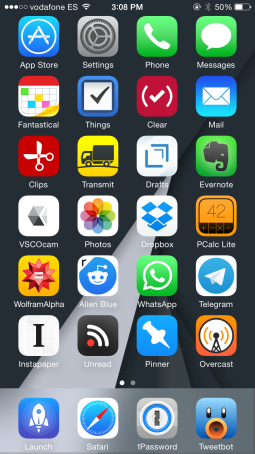**Descriptive Caption:**

The image showcases the phone's settings page, featuring a minimalist design. At the top left corner, the screen displays five dots—three filled-in on the left and two hollow on the right—indicating the current page within a series. The top section of the screen has a dark, sparkly gray background with "E5" in white text. To the right of this text lies a Wi-Fi symbol.

The middle of the top bar shows the current time, 3:08 PM. Adjacent to the time are icons for a Bluetooth connection and battery status, which is at 50% capacity with the battery icon half-filled in white.

The main section of the screen contains a grid of 24 app icons arranged in a 4x6 layout. The listed apps, in top-to-bottom, left-to-right order, are: 
1. App Store 
2. Settings 
3. Phone 
4. Messages 
5. Fantastical 
6. Things 
7. Clear 
8. Mail 
9. Clips 
10. Transmit 
11. Drafts 
12. Evernote 
13. VSCO 
14. Camera 
15. Photos 
16. Dropbox 
17. PC 
18. Calc 
19. Light 
20. Wolfram Alpha 
21. Alien Blue 
22. WhatsApp 
23. Telegram 
24. Instapaper 
25. Unread 
26. Pinner 
27. Overcast.

The navigation bar at the bottom of the screen features three main icons—Launch Safari, 1Password, and Tweetbot—over a slightly transparent overlay. The overall background of the phone's screen is a lighter gray tone with a minimalist, triangle-based swirl design in the center, adding a subtle yet stylish touch.